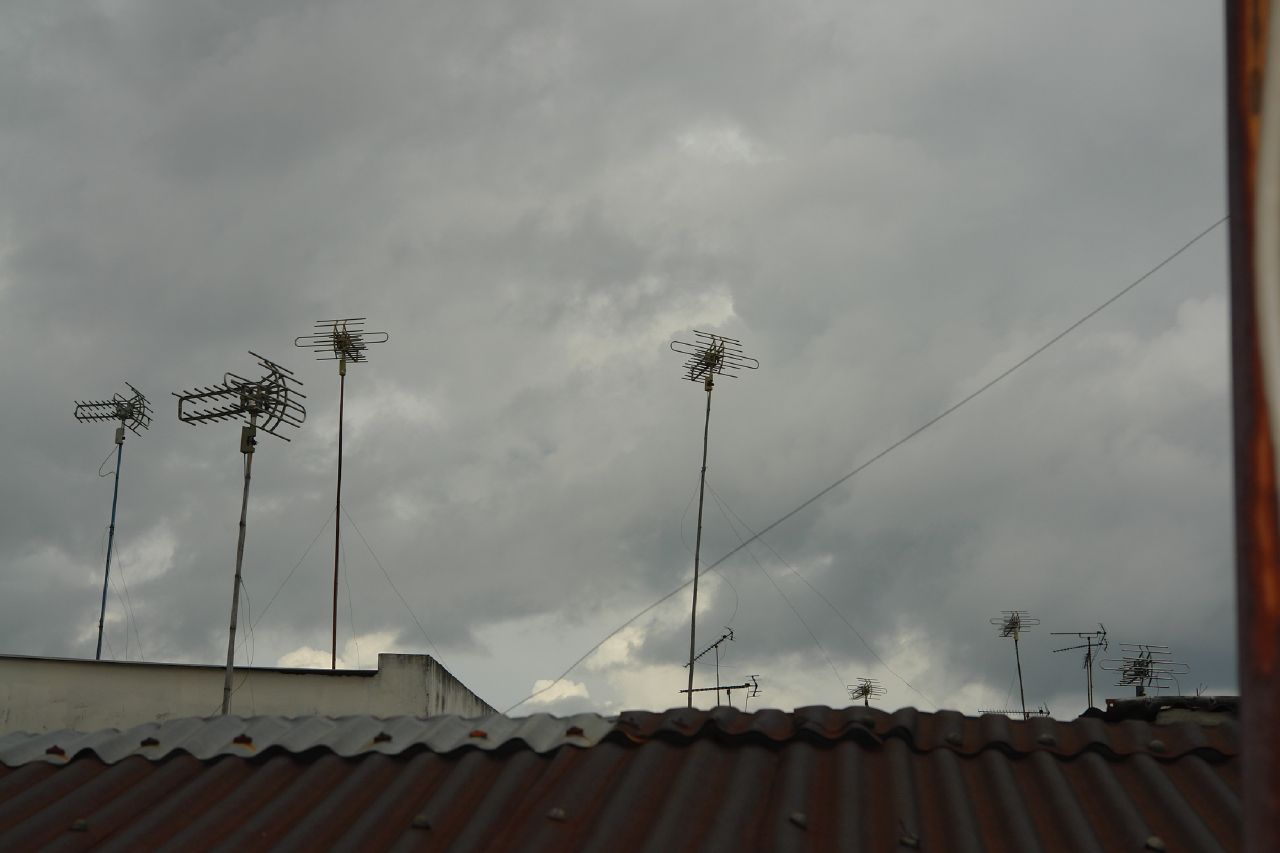The image shows the rooftop of a business building captured outdoors. The sky, covered in dark gray clouds, suggests imminent rain, creating an overcast and hazy atmosphere with minimal sunlight peeping through. The roof itself is characterized by wavy vertical ripples and features a dark gray color with a silvery section in the upper left corner. The building’s architecture includes a mix of metal and copper-brown tones with discernible vertical lines. Multiple antennas and poles, resembling light poles, protrude from both this roof and an adjacent roof of an old off-white cream-colored building visible on the left. These poles have various attachments, and several electrical wires crisscross the sky, with one prominent wire stretching diagonally from the right to the lower middle of the photo.